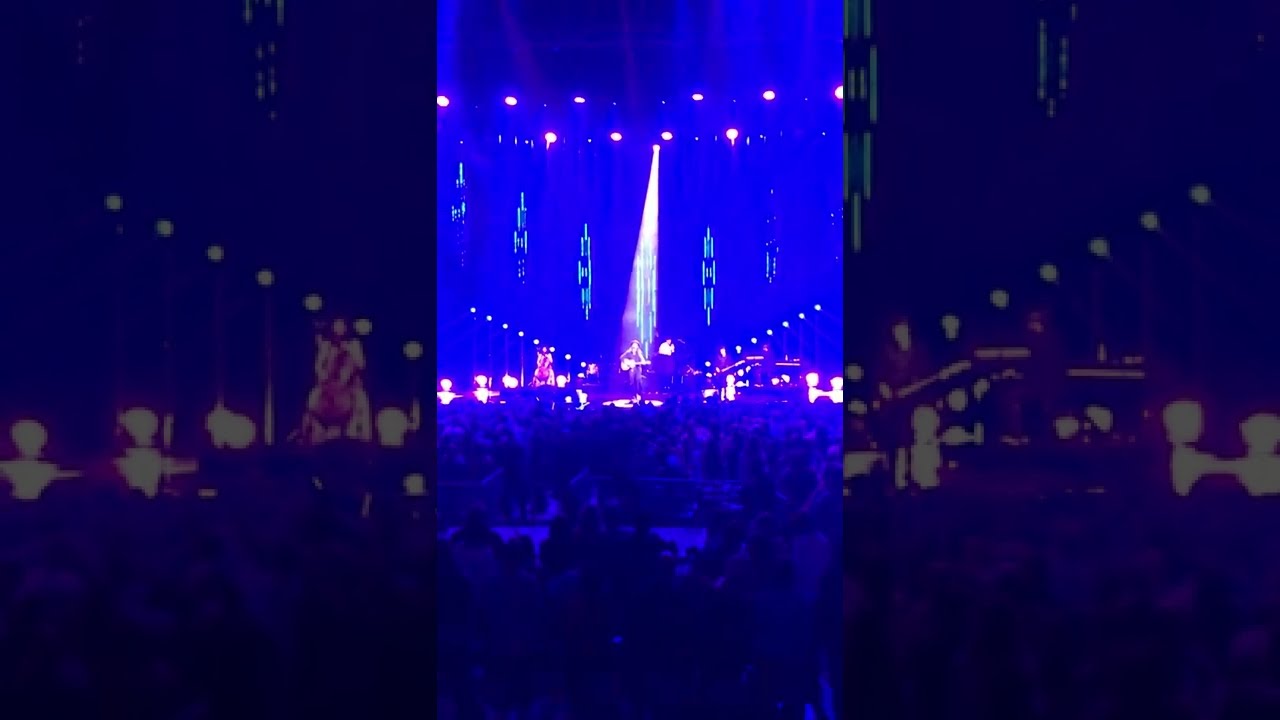The image captures a vibrant concert scene with a blue-hued atmosphere and bright stage lighting that highlights the performers. At the center of the stage, which is flanked by dark side screens, multiple musicians are positioned under spotlight beams originating from above. The stage features a diverse array of instruments, including a guitar, drum set, organ, and possibly a cello. There are at least two guitarists, with the main performer also appearing to hold a guitar. The background of the stage is predominantly blue with lavender lighting accents enhancing the setting. Below the stage, a large audience, partially visible and illuminated minimally, is seen from the back, cheering and enjoying the performance. The seating is organized into sections with railings and walkways. The performers are predominantly male, and the entire scene is suffused with a blue haze, creating a dynamic and immersive concert experience.